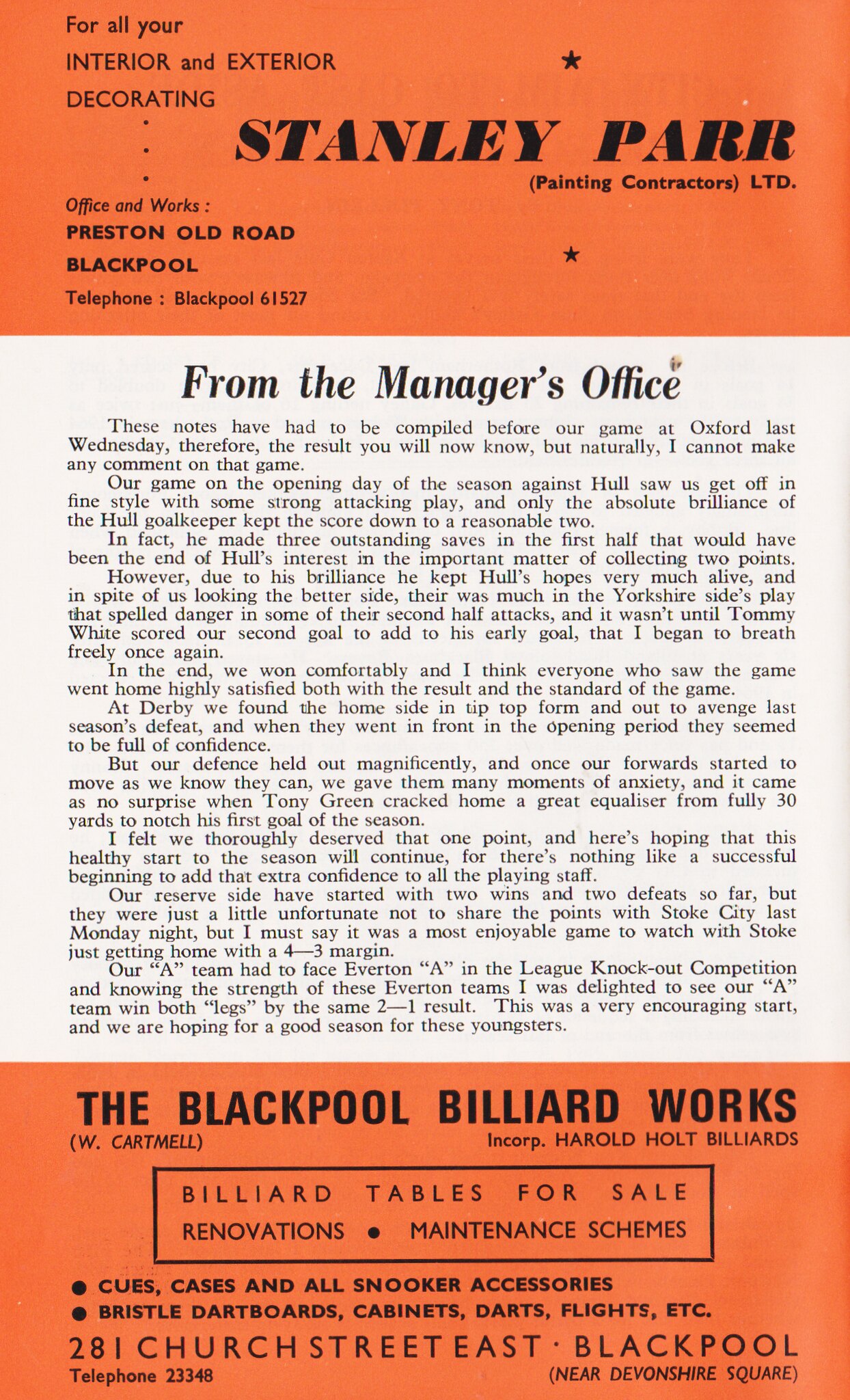The image features a program note, likely from a soccer team, with a prominent advertisement for Stanley Parr Painting Contractors Ltd., located at Preston Old Road, Blackpool. The text is displayed with an orange background and black lettering in the header and footer, while the manager's note appears on a white background with black text. The manager's note discusses preparations before a game at Oxford, mentioning that the results are known but no comments can be made. It also reflects on a previous game against Hull, highlighting the team's strong attacking play and the impressive performance of Hull's goalkeeper. Below the manager's note, there's an advertisement for Blackpool Billiard Works offering billiard tables for sale alongside renovation and maintenance services. The overall style suggests this is a page from a soccer team's program.